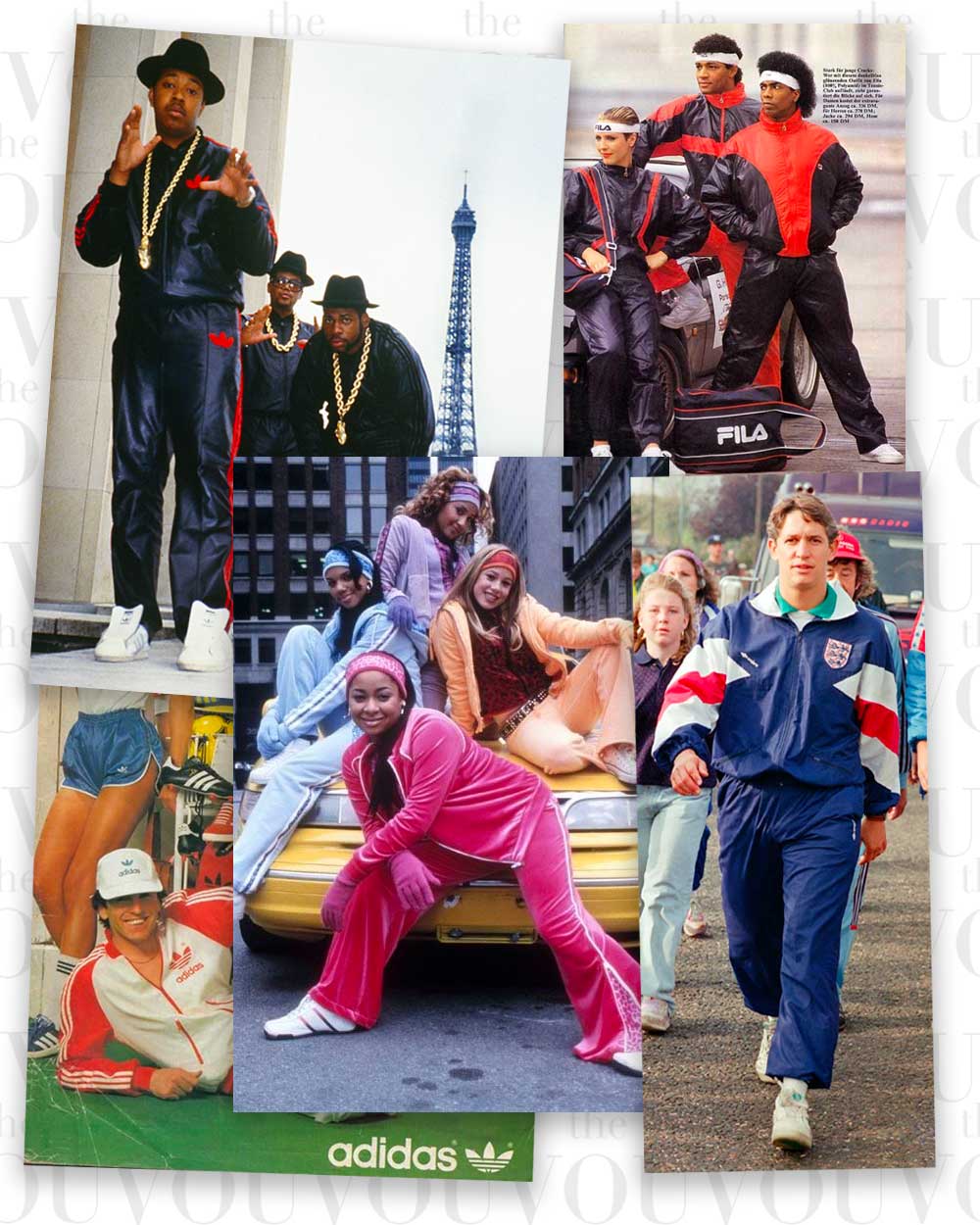This collage consists of five photographs showcasing individuals in street gear, some of whom are celebrities. The top left image features the iconic members of Run DMC, adorned in heavy gold chains and blue track suits, striking a pose in front of the Eiffel Tower. Moving to the top right, three athletes, two men and a woman, are dressed in red and blue track suits with white headbands, and a Thilo logo is evident at the bottom of this image. The center photo captures the actor from "That's So Raven" along with three other teen female stars, all seated on a taxi in what appears to be New York City, donning early 2000s suede sweatsuits. In the bottom right, a white male in a blue track suit walks toward the camera, surrounded by a crowd. The final image, partially obscured and tucked behind others, shows a white male in a white and red track jacket, lying down with a white cap, and behind him, the lower half of a female figure in blue running shorts and white crew socks. The bottom of this partially seen photo includes a green bar with the old Adidas logo. These images collectively display a blend of street fashion, featuring both Adidas and other brands, against backdrops ranging from Paris to New York. The collage also bears a faint repeating watermark at the bottom, displaying the characters "V.O.U." in gray.